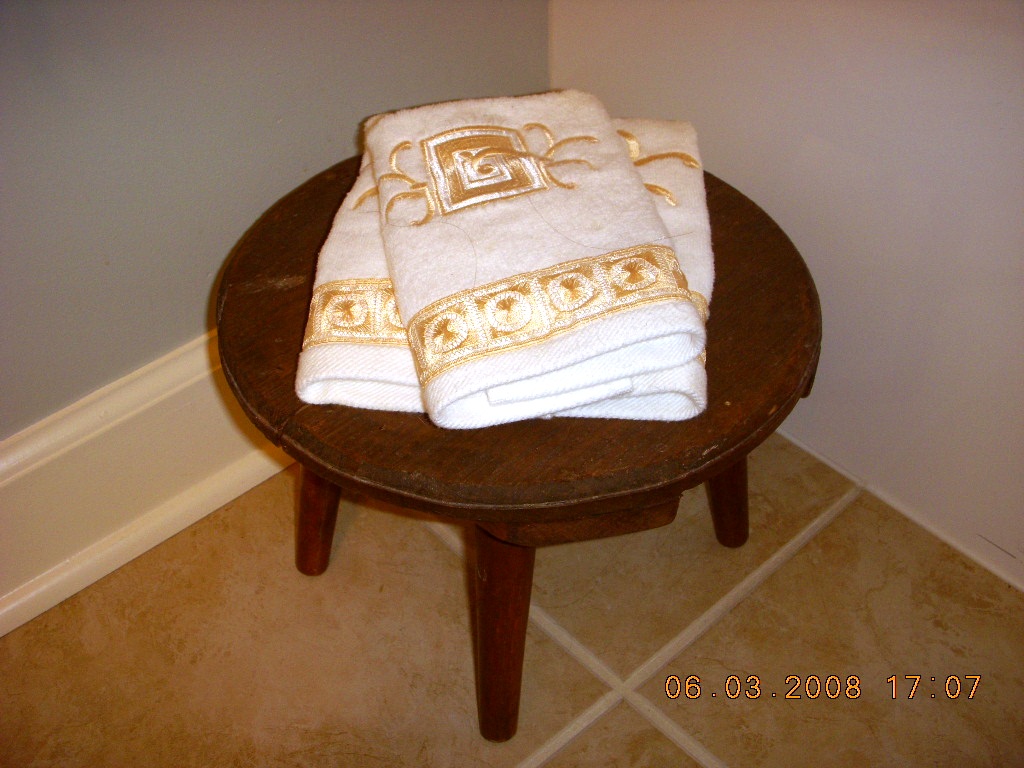In the photograph, a cherry-brown wooden stool, possibly an end table, is positioned in the corner of a room. The stool has three visible peg legs, with the possibility of a fourth leg that is obscured from the top-down perspective. Resting neatly atop the stool are one or two white folded towels, adorned with gold embroidery along the edges and a gold emblem at the center.

The room reflects a potentially intimate space like a bathroom or kitchen, characterized by its gold-hued tile flooring set with beige or cream-colored grout. The corner placement of the stool reveals two walls meeting at an angle: the left wall is painted a light blue and features white crown molding along the base, while the right wall appears plain white without any molding.

In the bottom right-hand corner of the image, the date and time "06-03-2008 at 17:07" are displayed in a digital text format, further grounding the setting in a specific moment.